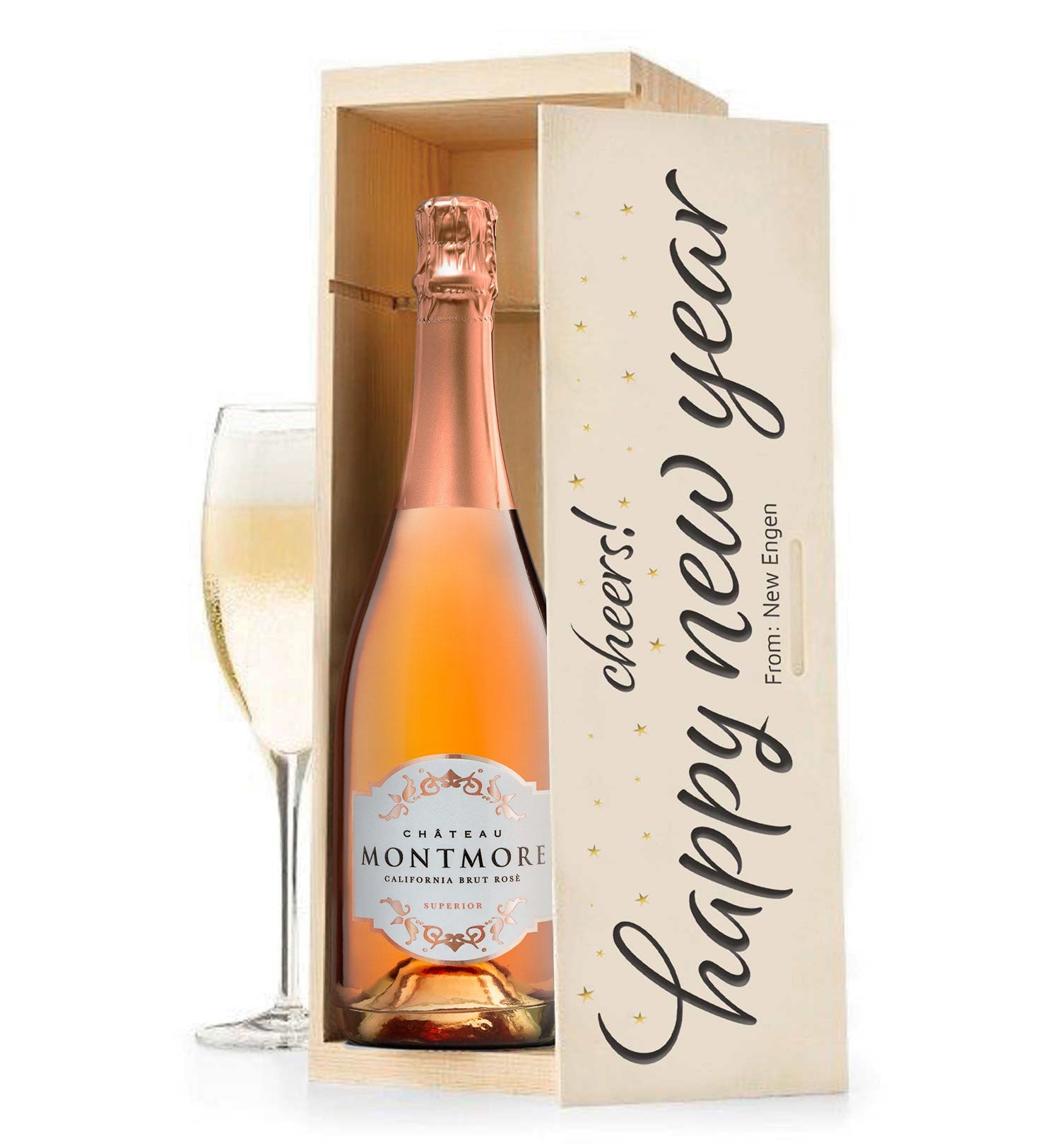This product image showcases a bottle of pink-colored champagne resting inside an open cedar gift box. The lid of the box, which is positioned to the right, features a festive message in black cursive text surrounded by small yellow stars: "Cheers! Happy New Year from New Engen." The bottle itself is adorned with a rose gold foil on top and has a white label with rose gold accents, stating "Chateau Montmore, California, Brut Rosé, Superior." To the left of the box sits a champagne glass filled with the bubbly beverage, crowned with a large, frothy head.